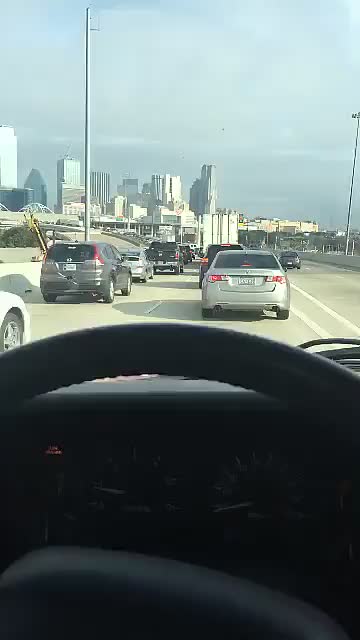This photograph, seemingly taken from the driver's seat of a car, captures the view through the front windshield of a busy four-lane interstate leading towards the downtown area of a city with numerous skyscrapers on the horizon. The overcast sky casts a bright but diffused light over the scene, in contrast to the dark interior of the vehicle where the dashboard, steering wheel, speedometer, and a lit check engine light are visible. Traffic is dense, with many cars ahead, including a silver car directly in front and a truck two vehicles ahead. To the right, there is an exit lane that is less congested. The downtown area is situated towards the left of the horizon, while the right side remains more open. There is also an impression of potential roadwork on the left lanes, contributing to the traffic congestion, suggesting a scene of halted or slow-moving traffic on a metropolitan highway.